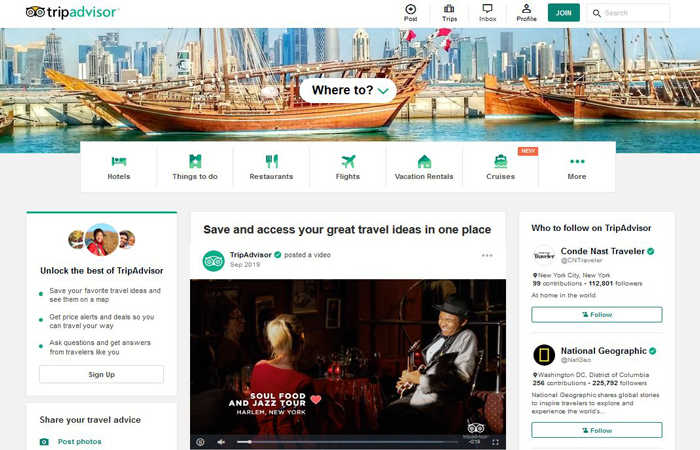The screenshot portrays the desktop version of the TripAdvisor website. Dominating the top portion is a large banner showcasing vintage wooden ships docked at a bustling pier in what appears to be a downtown area. Below the banner, multiple sections are clearly visible, including "Hotels," "Things to Do," "Restaurants," "Flights," "Vacation Rentals," and "Cruises."

In the middle of the page, there's an embedded video featuring an interview with a jazz musician, part of the "Soul Food and Jazz Tour" in Harlem, New York. The overall background of the site is a light gray, complemented by numerous green elements that provide a cohesive and vibrant look.

The familiar TripAdvisor logo, characterized by owl eyes that resemble binoculars, is prominently displayed throughout the page. At the top right, users can find a search bar and a green "Join" button for account sign-up. The site also features social media links under a "Who to Follow" section, listing notable accounts like Condé Nast and National Geographic.